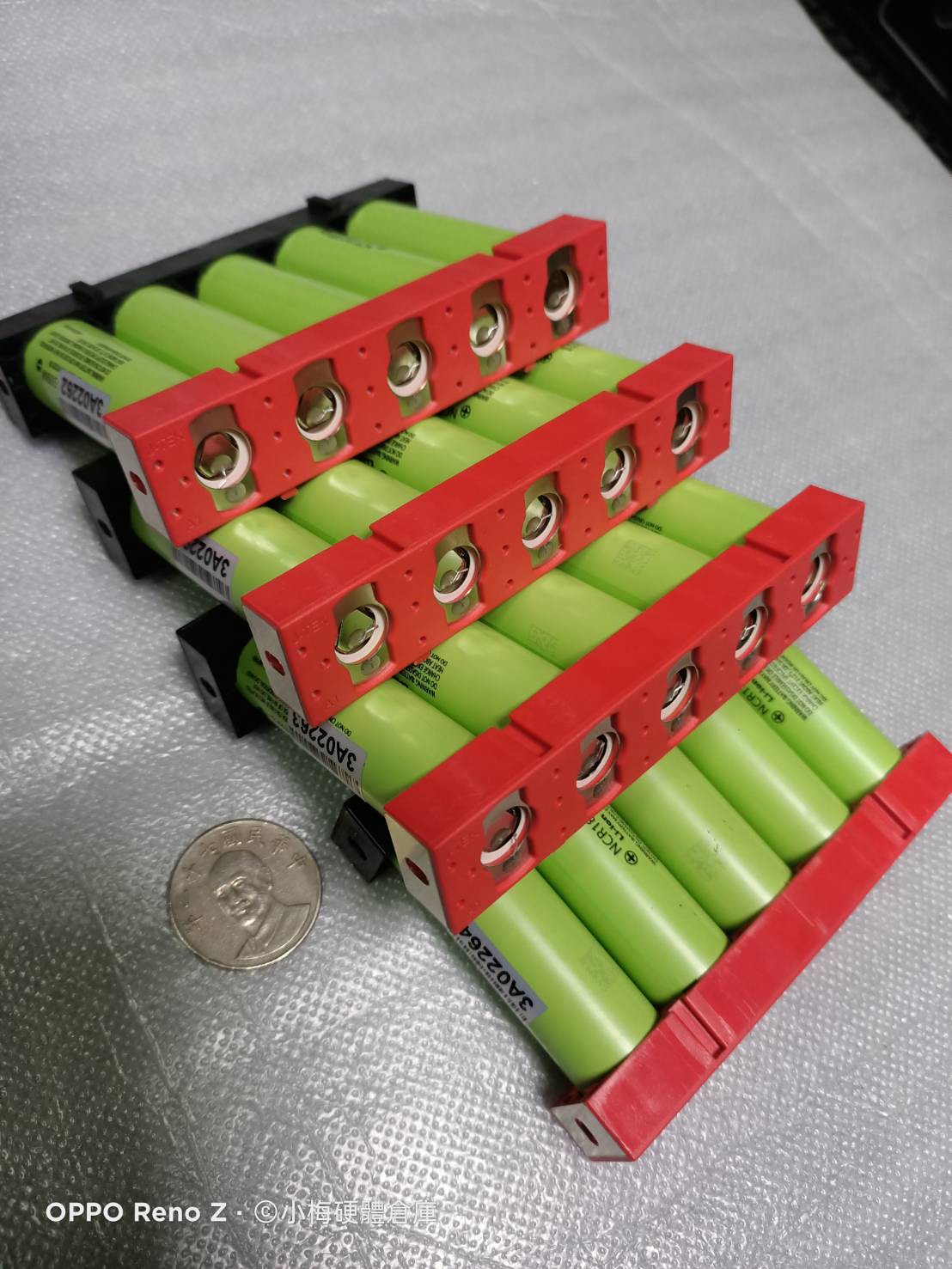This photograph features a set of green cylindrical objects that appear to be lithium-ion battery cells, potentially similar to 18650 batteries but somewhat unique in their dimensions, being slightly shorter and wider. The batteries are lime green and each bears the label "3A02263" or "02264," potentially indicating their serial numbers. Positioned beside the batteries for scale is a coin, possibly Chinese, providing context for their size, which is approximately two to two and a half coins in length.

These batteries are neatly arranged within a frame-like structure, secured between a red bar at the bottom and a black bar at the top. The bottom of each green tube extends slightly through the red bar, with holes in the red section displaying a silver color. The setup appears to be drawing power from the batteries in series, although the exact purpose is unclear. The entire assembly is laid flat on a semi-transparent tarp, and there is also text reading "OPPO RENO Z" visible in white, likely related to the device or surface on which the components rest.